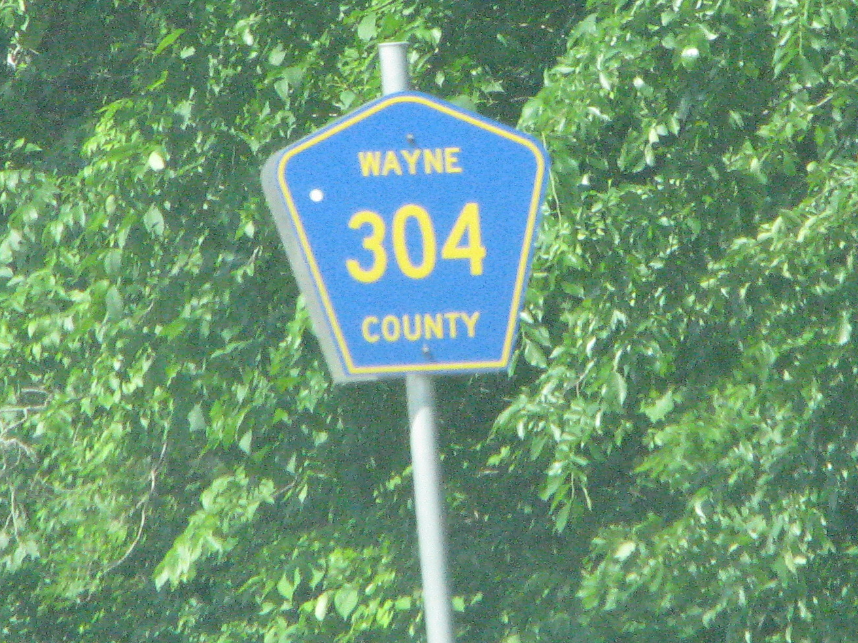In this somewhat grainy photo taken during a bright, sunny afternoon, a close-up view captures a uniquely shaped street sign mounted on a metal tubular pole. The sign resembles a king's crown or a chef's hat, with a narrow base that broadens as it extends upward before coming to a rounded peak. Its vivid blue surface is contrasted by bold gold lettering that reads "Wayne," followed by the number "304," and below that, "County." Behind the sign, a dense thicket of tree branches and leaves dominates the background, creating a lush tapestry of vibrant green foliage illuminated by the strong sunlight. The trunks and limbs of the trees are obscured, leaving an impression of abundant greenery basking in the afternoon sun.